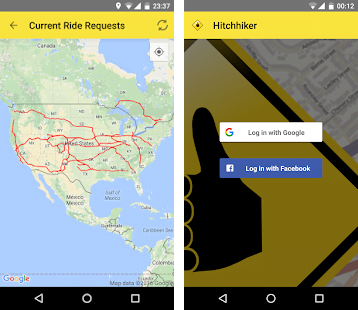The image features two portrait-oriented screenshots placed side by side, bordered by a thin white line, creating a nearly square overall composition. Each screenshot, rectangular and approximately twice as tall as they are wide, seems to be captured from a cell phone given their standard proportions.

The left screenshot has a grey top border displaying various status icons: a navigation pin, a half-full WiFi signal, a fully connected network bar, a half-filled vertical battery icon, and the time reading 23:37. Below this is a horizontal yellow banner with a left arrow icon, the text "Current Ride Requests," and a map of the USA with red squiggly lines, likely depicting routes.

The right screenshot, slightly different yet similar in layout, shows a marginally lower WiFi meter, a fully connected network bar, a half-filled vertical battery icon, and the time reading 00:12. It also features a yellow banner with the text "Hitchhiker" and a yellow diamond icon with a black symbol inside. The background includes an image of a thumbs up inside a yellow diamond with a black border. Below this are two login options: a white box labeled "Log in with Google" and a blue box labeled "Log in with Facebook."

Overall, the image captures detailed aspects of two mobile app screens adjacent to one another, illustrating different time-based states and components of the app interface related to ride requests and hitchhiking.